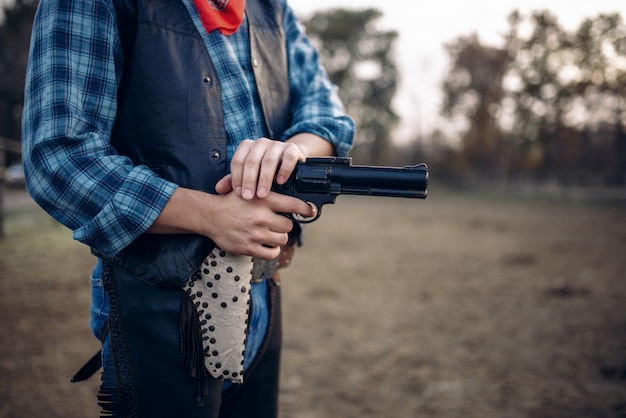In the image, we see a man dressed as a cowboy, standing outdoors with a backdrop of blurred, tall trees and a mix of dirt and dying, brownish-gray grass. The cowboy is seen from the neck down, clad in a dark blue vest over a blue plaid button-up shirt with rolled-up sleeves exposing his forearms. Around his neck, a red bandana is knotted, and he wears blue jeans paired with black chaps. His gun holster, stitched together with a distinct tan color and adorned with black spots or studs, holds a black revolver. The man grips the gun with both hands: his right hand is firmly wrapped around the handle inside the trigger guard with his index finger resting near the trigger, and his left hand is placed over the hammer, suggesting he is ready to fan it back for rapid fire. The ground beneath him is a mix of dirt and grass, emphasizing the outdoor setting.